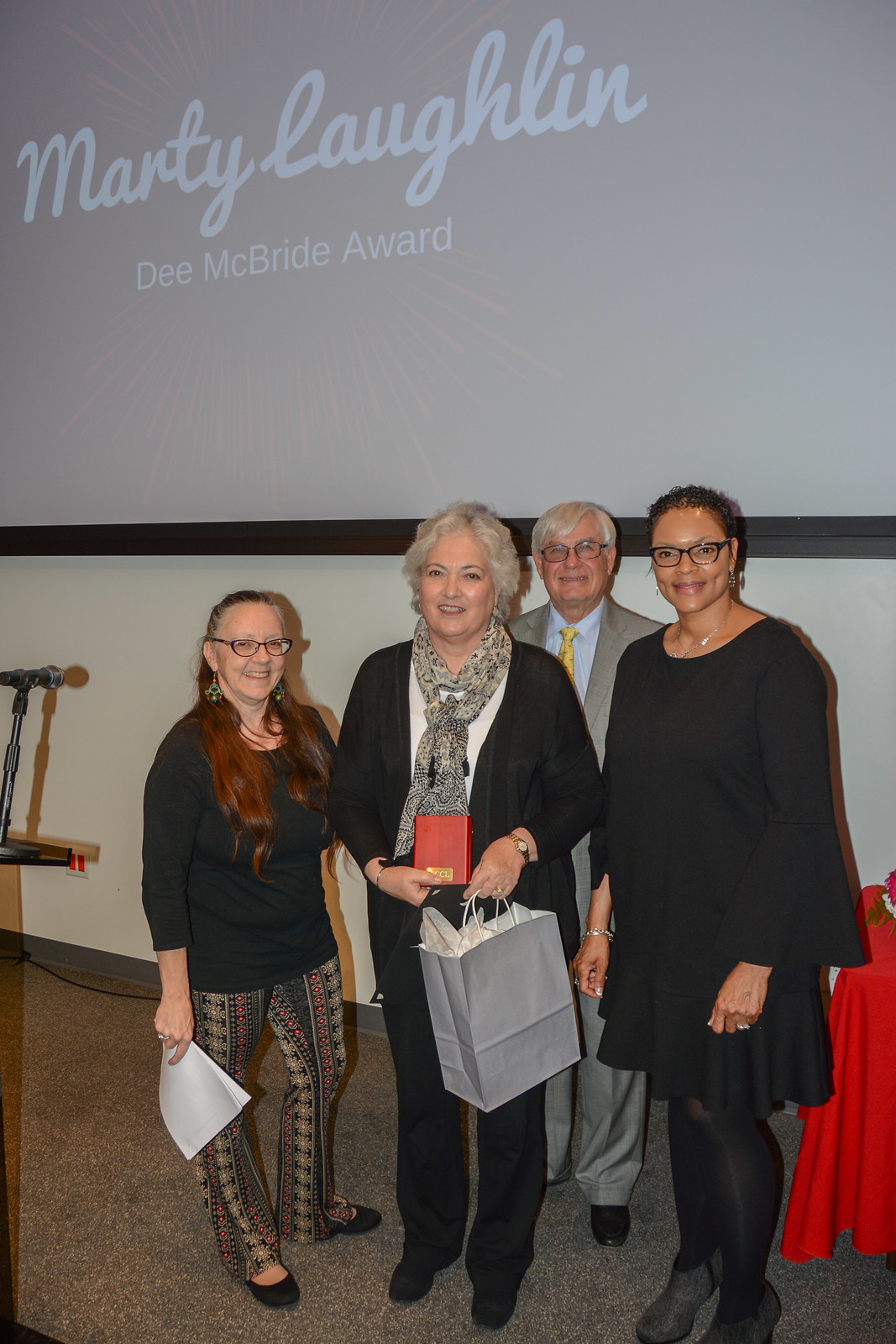In the photograph, four people are standing together beneath a sign that reads "Marty Laughlin D. McBride Award." The group consists of three women and one man, all dressed in business professional attire. In the front, a woman with silver hair, dressed in a black pantsuit and a gray scarf, holding a gray gift bag, stands centrally. Behind her, a man with white hair, black glasses, and a beige suit paired with a blue shirt and a yellow tie, positions himself. On the left, a shorter woman with long red hair and glasses wears a black top and multicolored, paisley-patterned pants; she holds a stack of papers in her right hand. On the right, another woman is dressed completely in black—including her dress, tights, shoes, and glasses—standing beside the edge of a table draped with a red tablecloth. The setting appears to be indoors, featuring a large screen in the background displaying the award’s title.